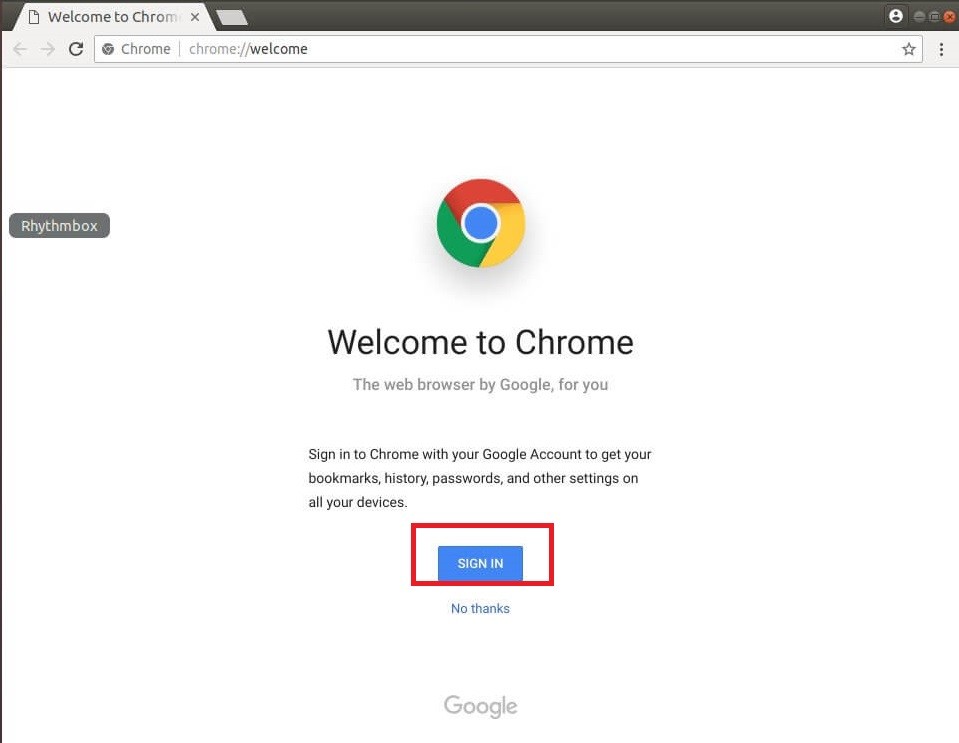This detailed caption can be refined and expanded as follows:

---

This image is a screenshot of a web browser page displaying Google Chrome. At the very top of the interface is a dark grey header. On the left side of this header, there's a light grey tab with angled left and right edges. Inside the tab is faded dark grey text that reads "Welcome to Chrome." This text gradually fades out to light grey towards the right end of the tab, where a dark grey 'X' icon is situated. To the far left of this tab, there's a dark grey icon of a piece of paper with its top right corner folded over.

Beneath the header, the navigation bar begins with a series of control icons. These include a light grey arrow pointing left (back button), a light grey arrow pointing right (forward button), and a black refresh icon (reload button). To the right of these controls is a rectangular white URL bar. At the left end of the URL bar, there's a dark grey Chrome icon consisting of a dark grey circle with another dark grey circle inside it, surrounded by white radial outlines. Next to this, dark grey text reads "Chrome."

Following the "Chrome" text, there is a light grey vertical separator. To the right of this separator, in light grey text, it reads "chrome://" followed by black text that says "Welcome." Towards the far right end of the search bar, there is a dark grey star icon, which typically indicates a bookmark option. Outside and to the right of the URL bar, there are three dark grey dots stacked vertically representing the browser menu or options.

Below the navigation bar is the body of the page, which has a white background. On the left side of the page, there is a dark grey rectangle with rounded corners and white text inside that reads "Rhythm Box." Centered at the top of the main body of the page is another Chrome icon, this time in its full color scheme: green on the bottom left, red on the top, yellow on the bottom right, and a blue circle in the center. This colorful Chrome icon casts a light grey shadow onto the white background.

Below the colored Chrome icon, there is prominent, enlarged black text that says "Welcome to Chrome," with additional, smaller text underneath providing further information or instructions.

---

This caption provides a comprehensive and structured description of the browser page screenshot.